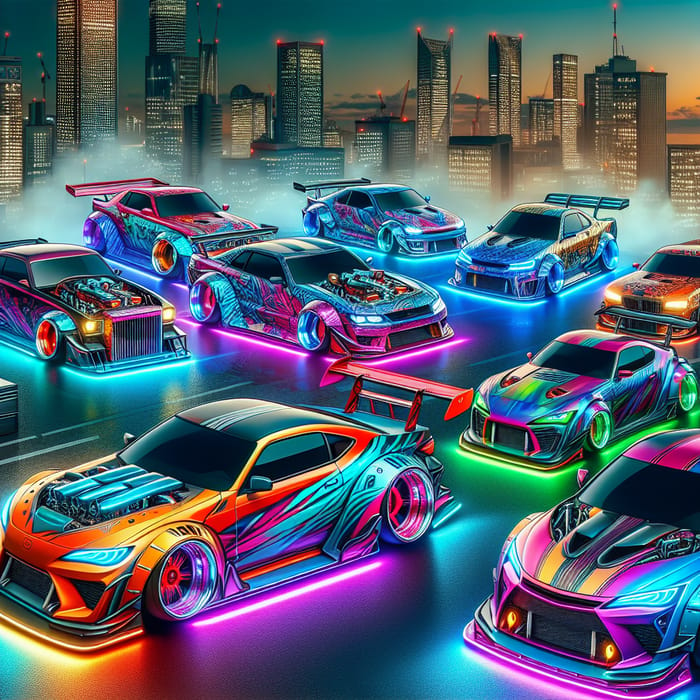This vibrant, square-format digital graphic showcases a collection of lowered race cars, each adorned with neon glowing lights underneath. These cars, likely from Asian manufacturers such as Nissan and Toyota, are illustrated in a distinctive neon art style. All the race cars are equipped with tail spoilers attached to their trunks, enhancing their aerodynamics to minimize drifting.

In the foreground, two rows of cars face the bottom left corner of the image, with the nearest vehicles glowing neon pink and orange. Behind them, a car shines in neon green, followed by another in neon orange, and two more in neon blue. At the midpoint along the left side, several cars face the right, each illuminated with vibrant neon pink, while on the far left, a roadster-type vehicle glows aqua.

Set against a shimmering, glass-like road surface, these cars are backed by a striking city skyline filled with towering skyscrapers, further highlighting the dynamic and electrifying atmosphere of this detailed and colorful illustration.